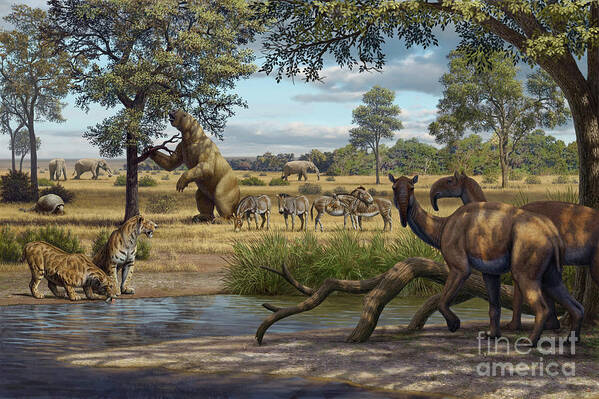This highly detailed and intricate illustration from Fine Art America depicts a vibrant prehistoric scene set in a desert-like landscape with lush, verdant trees on the right-hand side. A diverse array of animals is scattered throughout the scene, drawing the viewer into a bustling ecosystem.

On the left side, saber-toothed tigers and a large bear standing on its hind legs reach up for leaves from a nearby tree. Nearby, zebras or antelope-like creatures mingle in the central area, not far from a watering hole where the saber-toothed tigers are drinking. The foreground features elephants grazing in the background, their presence the only nod to contemporary wildlife within this otherwise ancient tableau.

Adding to the diversity, peculiar long-snouted creatures resembling a blend of anteaters and elks are seen resting under the shade of trees near the water. Among these prehistoric inhabitants is also a shelled creature in the distant background. The image is not just a random assortment but a well-organized artwork capturing an imagined prehistoric milieu, down to the fine details and the animating style that brings the scene to life. The bottom right-hand corner of the illustration is marked with "Fine Art America" in white lettering.